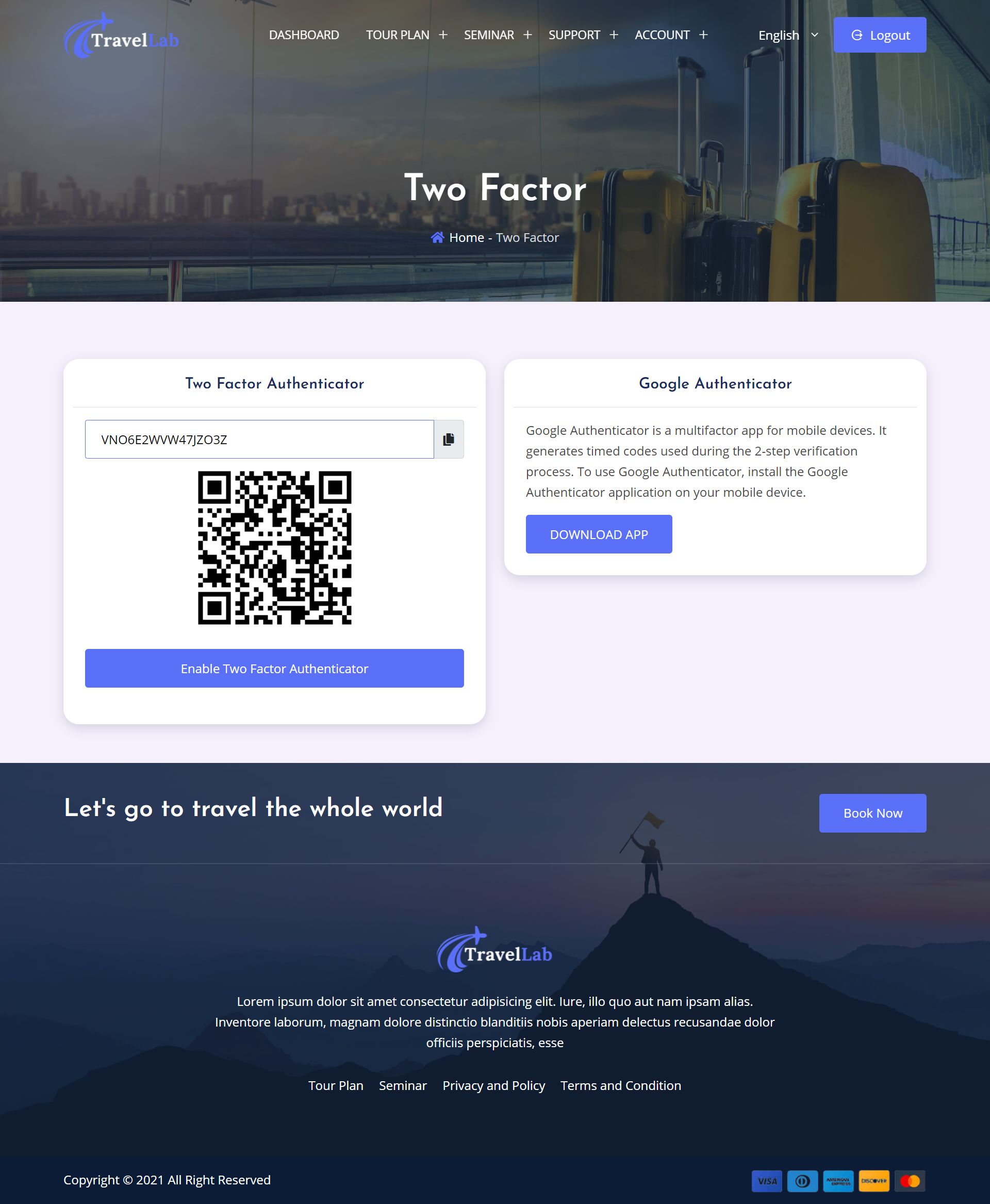The image features a travel-related user interface design for an application called "Travel Lab." At the top left, the "Travel Lab" logo is displayed, with "Travel" in white and "Lab" in blue. An icon of a blue airplane with a trailing blue line accompanies the text. The top section of the interface includes white text tabs labeled "Dashboard," "Top Land," "Seminar," "Support," "Account," and "English." Positioned on the top right is a blue "Log Out" button.

In the center of the image, white text reads "Two-Factor Home" and "Two-Factor." On the right side of the background, there are yellow suitcases with a black one in the middle, situated in what appears to be an airport setting. Visible through the windows in the background are various buildings.

Below the main image area, on the left side, detailed instructions for setting up a two-factor authenticator are provided. The text "Two-Factor Authenticator" is followed by a field for entering an authentication code, which is displayed as VN06A2VW47JZ03Z. A black QR code is located below this field, alongside a blue "Enable Two-Factor Authenticator" button.

On the right side, information about "Google Authenticator" is given. The description explains that Google Authenticator is a mobile application used for generating time-based codes during the two-step verification process and provides instructions for installing it on a mobile device. Below this information is a blue "Download App" button.

The bottom section of the image features a purple background with a black mountain graphic, showing a person raising a flag at the mountain's peak. The white text reads "Let's go travel the whole world," and a blue "Book Now" button is positioned to the right. The bottom left corner repeats the "Travel Lab" icon and includes additional text in a different language, with tabs underneath labeled "Top Line," "Seminar," "Privacy and Policy," and "Terms and Conditions." In the bottom right corner, payment options are displayed, showing the logos for MasterCard and Visa, with three other options not visible.